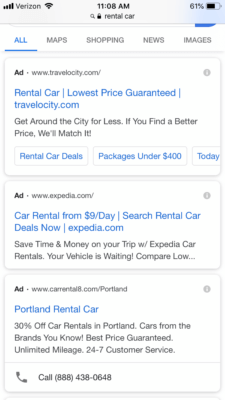The image is a screenshot from a smartphone displaying a web search result for "rental car." At the top of the screen, the status bar indicates full signal strength with four bars on the left, the word "Verizon" in the center, the time "11:08 a.m." displayed next to it, and a battery icon showing 61% charge on the right. Below the status bar, a search query for "rental car" is visible alongside a search button, followed by a navigation bar with the options: "All" (highlighted in blue and underlined), "Maps," "Shopping," "News," and "Images."

The webpage appears to show multiple advertisements for rental cars. The first ad, marked by a small "Ad" icon and linked to Travelocity.com, advertises "Rental car, lowest price guaranteed." It highlights benefits such as getting around the city for less and price matching guarantees.

The second ad, also marked as an advertisement, promotes Expedia.com, offering car rentals starting at $9 a day and encouraging users to "search rental deals now."

The final ad on the page is from carental8.com for Portland rentals. The ad features blue text that says "Portland rental car" and mentions a 30% discount on car rentals in Portland, featuring cars from well-known brands. It also emphasizes best price guarantees, unlimited mileage, and 24/7 customer service. There is an image of a phone with a caption instructing users to call 888-438-0648 for more information.

The screenshot provides a snapshot of various rental car options, showcasing different deals from major travel websites.